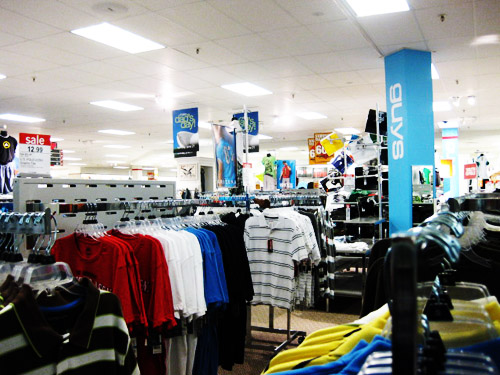This image depicts the interior of an unidentified clothing store with a modern retail design. The ceiling features a grid of drop tiles interspersed with black sprinkler heads and large rectangular fluorescent lights, ensuring the space is well-lit. On the left-hand side, approximately an eighth of the way in, a prominent blue column with the word "Guys" written vertically in white letters indicates a section dedicated to men's clothing. 

In the foreground, a variety of striped shirts and polos are prominently displayed, including a black and white striped shirt and several solid-colored polos in red, white, and blue, as well as a blue and white striped polo. To the left, partially visible, are some button-down shirts, recognizable by their exposed collars and shoulders.

Above the polos, a sale sign advertises a price of $12.99, suggesting a special offer or promotion. Additionally, the ceiling hosts signs celebrating Father's Day, reading "Dad's Day" in blue with yellow lettering. Towards the back of the store, a clearance section is indicated with signs announcing discounts of up to 60% off. The identity of the store remains unknown due to the absence of any visible branding or signage.